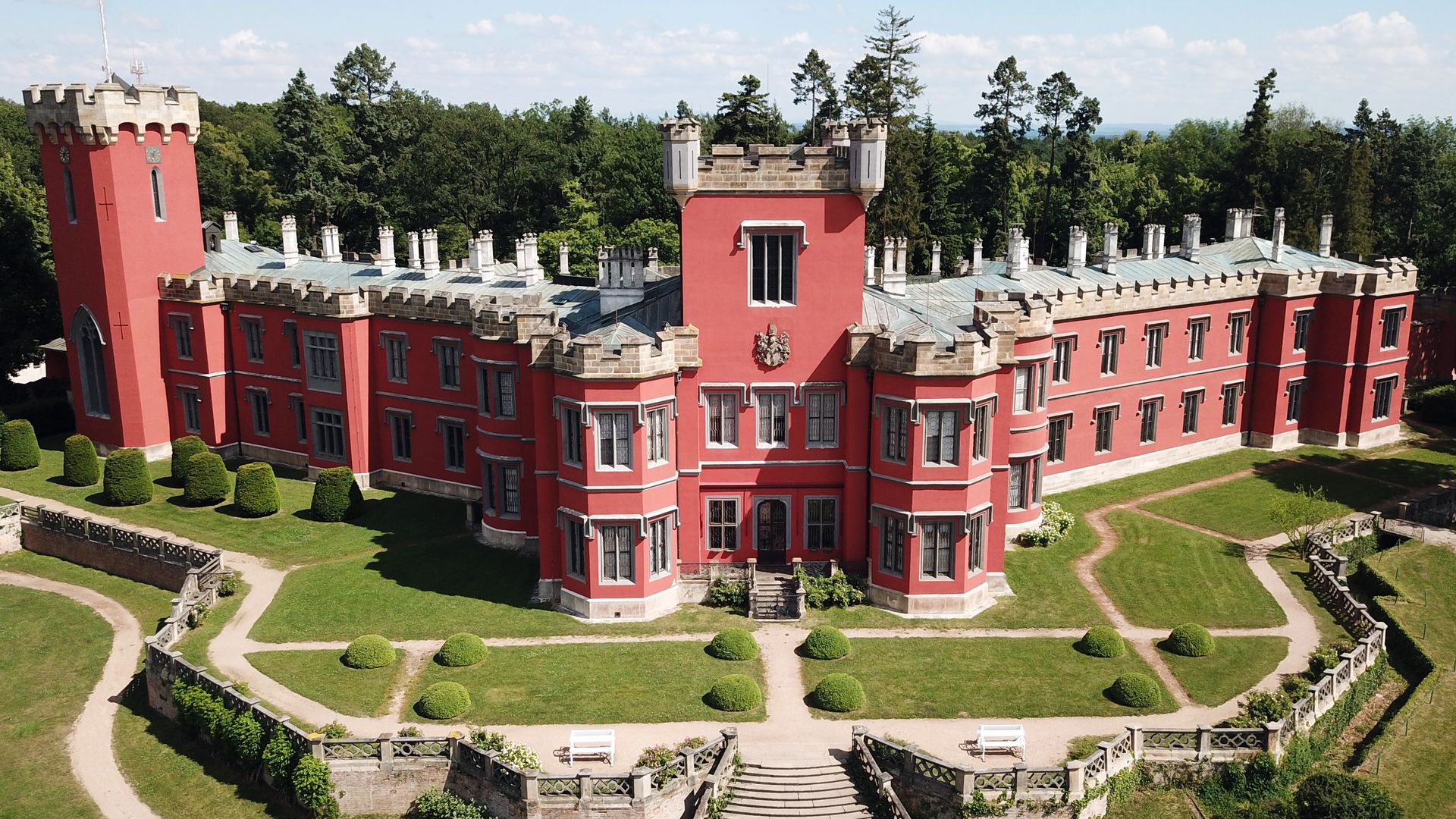The image is an outdoor scene showcasing a grand red palace with a distinctive white roof and multiple chimneys. The palace features a prominent three-story tower above the front door, adorned with an elaborate crest. The extensive landscaped front yard is meticulously maintained, featuring beautifully shaped shrubs, a neatly manicured lawn, and large concrete staircases leading up to the palace. Surrounding the palace is a concrete fence and pathways that weave through the greenery. In the background, a dense forest of trees stretches upwards, possibly against the backdrop of a distant mountain range. The sky above is blue and dotted with clouds, adding a picturesque quality to the overall view.